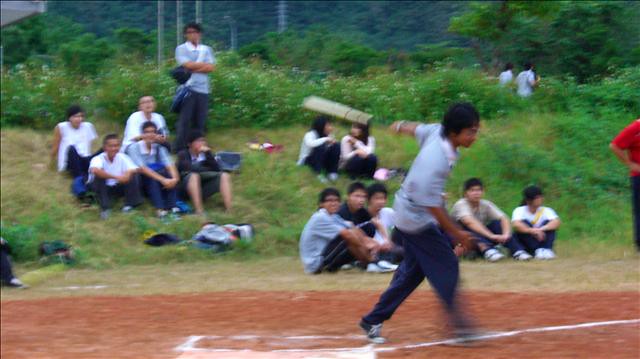This photograph, although slightly blurry, captures an outdoor scene of a baseball game in progress. The ground is a mix of reddish and tannish dirt, transitioning into a small green hillside and leading to a larger, darker green hill in the background. A prominent white stripe marks the sandy foreground, adjacent to a white rectangular shape that resembles a base. 

A male adolescent, dressed in long dark pants, dark shoes, and a light-colored shirt, is positioned near the base. His dark hair is noticeable as he stands sideways, bent slightly at the waist with his right arm crossing his body and his left arm extended behind him, as if in the act of throwing a ball or swinging a bat.

Behind him, sitting on the ground, are several spectators dressed in both dark and light-colored clothing. They are seated with their knees pulled to their chests and their forearms wrapped around their shins. Additional spectators are scattered on the hillside, observing the game in the same manner. Two girls on the right side of the hill appear to be engaged in conversation, while two more people are walking along the hill in the background. In the far right of the image, a man in a red shirt is also visible. The far distance reveals lush greenery of trees and brush, further framing this vibrant scene of recreational activity.